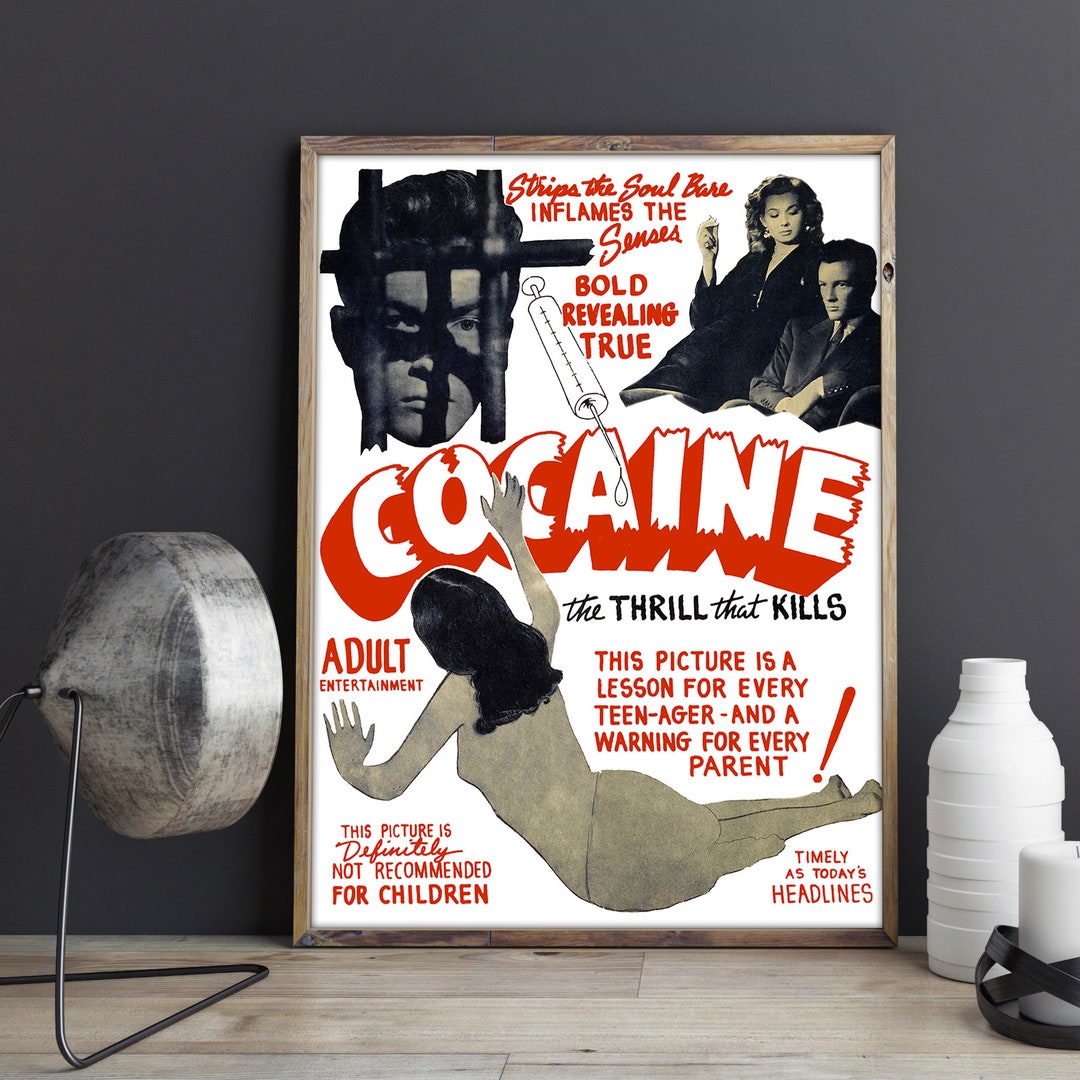In this photo, there's a framed, black and white movie poster for "Cocaine," set against a dark grey wall with a light wood floor. To the left of the poster, a spotlight casts a beam of light, while to the right, there are some canisters on the floor. The poster prominently features a variety of images and text. At the top left, a young man's face is seen behind jail bars. Directly to the right of this image, bold red text reads: "Strips the soul bare, inflames the senses, bold, revealing, true." Below these words, a large syringe with a dripping needle extends over the word "Cocaine," which is in white, outlined in red, giving a 3D effect. In the upper left-hand corner, the picture shows a man and woman engaged with each other, and in the middle, a woman is seen leaning on her hip with her back to the viewer. Another image depicts a woman appearing to overdose. Beneath the title "Cocaine," red text warns: "The thrill that kills." Following this, it states, "This picture is a lesson for every teenager and a warning for every parent," emphasized with a huge exclamation point. At the bottom right, it reads, "Timely as today's headlines," and to the left, "Adult entertainment" is highlighted in red. Finally, the bottom left corner concludes with the cautionary note: "This picture is definitely not recommended for children."